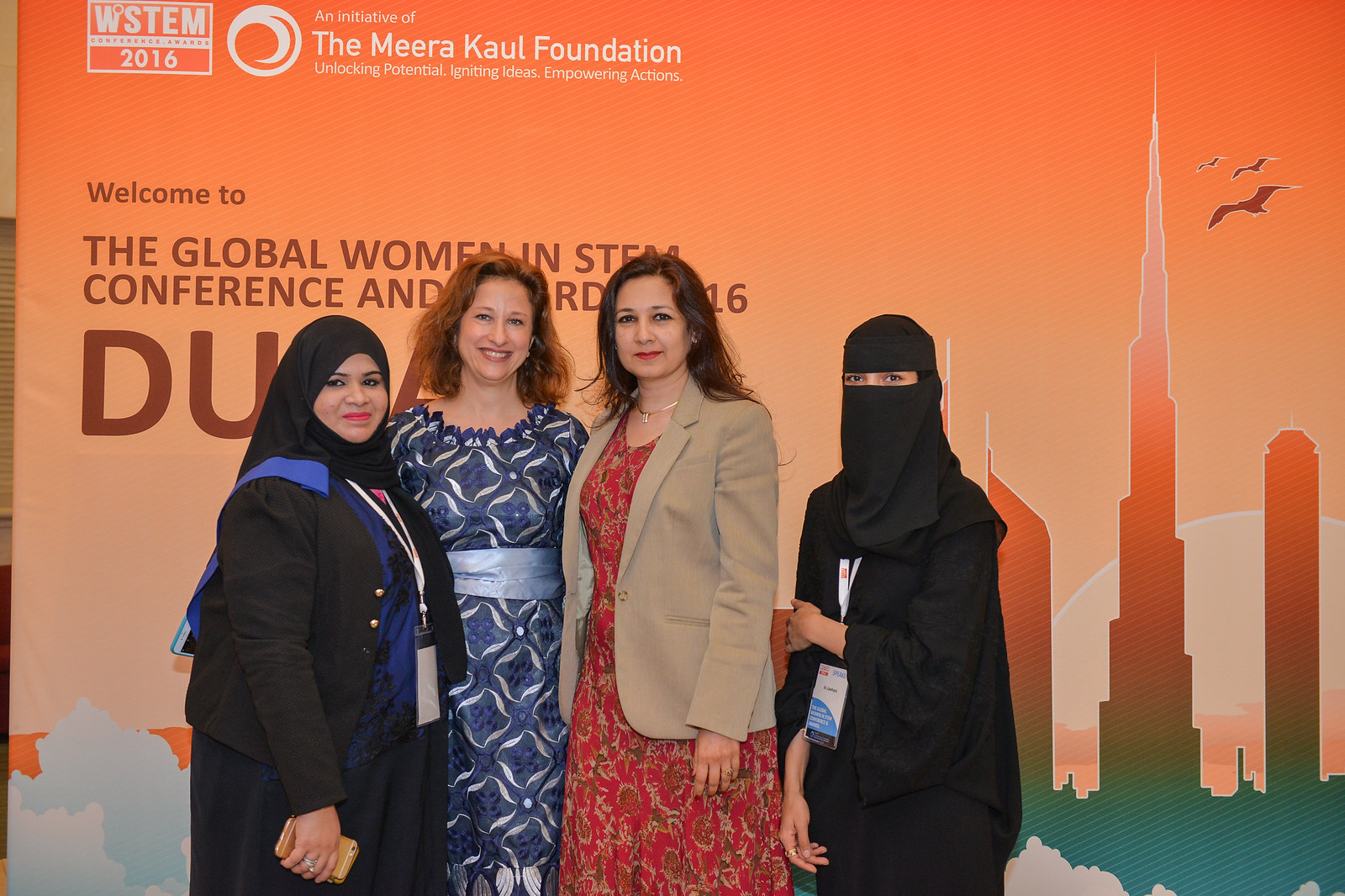This photograph captures four women standing in front of an orange backdrop at the "Global Women in STEM Conference, Dubai." The backdrop features the white graphic outline of the Burj Khalifa and text that reads, "Welcome to the Global Women in STEM Conference 2016" and "An initiative of the Miracle Foundation: Unlocking Potential, Igniting Ideas, Empowering Actions." 

Two women on the outer sides are wearing black burqas, with one of them (on the far right) also wearing a lanyard. The two women in the middle are dressed more casually: the woman on the center left is wearing a blue dress adorned with white patterns and a powder blue belt, and the woman on the center right is wearing a red dress with a design, paired with a tan blazer. Both of the women in the center have long brunette hair and are smiling at the camera, standing side by side with their companions, creating a juxtaposition of cultural attire against the vibrant and informative backdrop of the event.